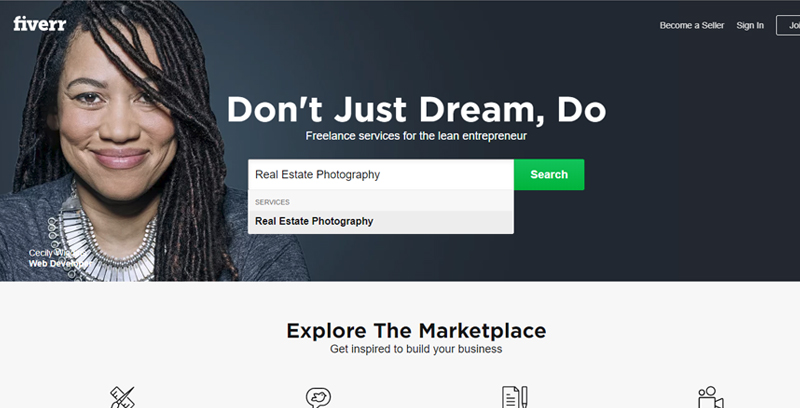This image is a promotional banner for the website Fiverr, designed to attract potential users and sellers. The design is centered around a navy-blue background, providing a professional and modern appeal. 

In the upper right corner, the navigation options are displayed in a clean white font, offering links to "Become a Seller," "Sign In," and "Join." Contrasting this, in the upper left corner, the bold white text prominently showcases the Fiverr logo, styled as "F I V E R R."

Prominently featured in the middle of the image is an inspiring call-to-action text in striking white font: "Don't just dream, do. Freelance services for the lean entrepreneur." Directly below this motivational message lies a practical search bar. The search bar, encased in a white box, is pre-populated with the text "real estate photography, services real estate photography." Adjacent to it, a green search button with white text instructs users to "Search."

On the left side of the image, there is a photograph of a smiling woman with long black dreadlocks. This image personalizes the banner and humanizes the platform, identifying her as "Cecillia, Web Developer.” 

At the bottom of the image, a gray banner stretches across the width, with the bold black text "Explore the marketplace" immediately catching attention. Below this, in smaller font, it encourages, "Get inspired to build your business." To support this call-to-action, there are four small icons beneath the text, representing various creative and professional services: a video camera, a paper with a pen, a bird inside a message bubble (likely symbolizing social media or communication), and a ruler crossed with a paintbrush.

Overall, this detailed and vibrant image effectively conveys Fiverr's value proposition, enticing users to engage with the platform.